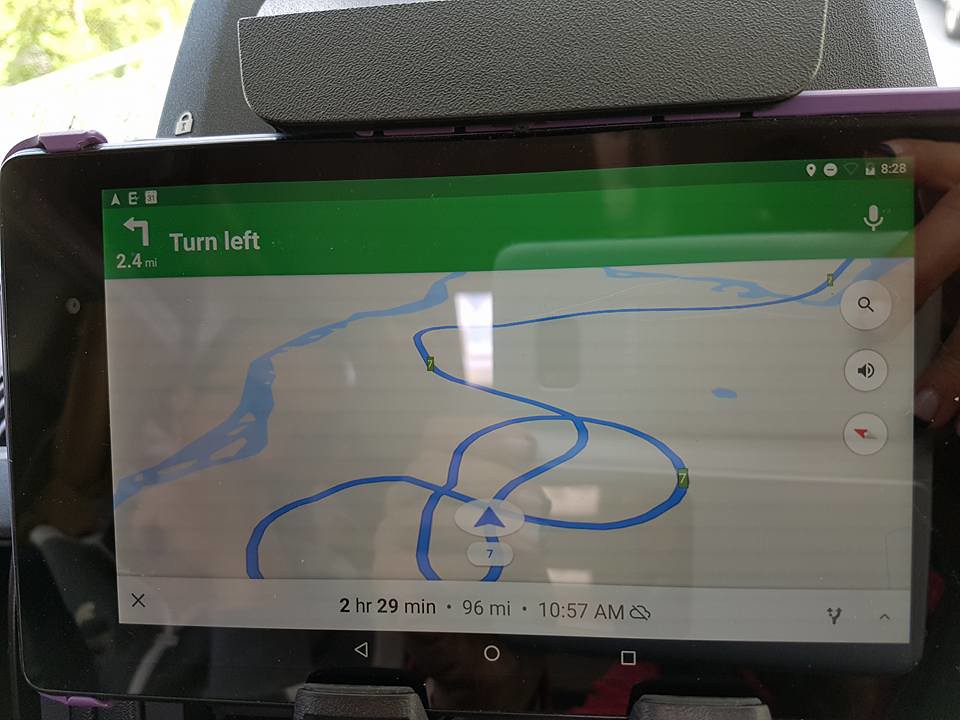This image captures a scene from inside a vehicle, focusing on a landscape-oriented screen, possibly a smartphone, securely mounted in a black clip just above it. The screen displays driving directions and a map, serving as a navigation aid. The screen is bordered in black with a distinctive green band running along the top. Within this band, an arrow points upwards and to the left, indicating a left turn in 2.4 miles, while a microphone symbol resides in the right corner. Above the green band, indicators for battery life, the time (8:28), Bluetooth, and other cellular information suggest the device is indeed a smartphone.

Peering out from the top left edge of the image, one can see light filtering through green leaves, as if viewed through the car's windshield. The map itself is predominantly white with twisty blue lines depicting the route. Two prominent dark blue paths crisscross the map, and to the left, a river winds up and off the screen. In the bottom left corner of the screen is an 'X', presumably to cancel the navigation. In the middle of the screen, information reads "2 hours, 29 minutes, 96 miles, 10:57 AM," providing travel duration, distance, and estimated arrival time.

Interestingly, the screen also reflects part of the car's interior, revealing a hand positioned towards the middle and an indistinct outline of a person's face to the upper left, adding a human element to this navigational snapshot.